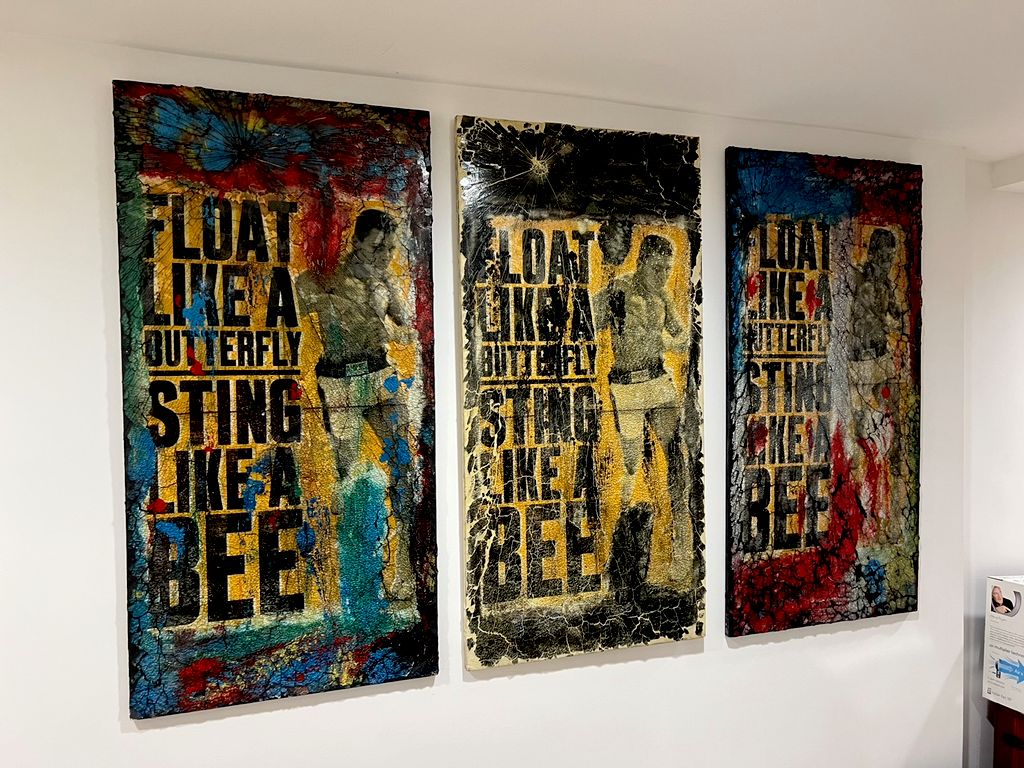This image captures a wall adorned with three distinct posters featuring the legendary boxer Muhammad Ali. Each poster showcases the same iconic quote, “Float like a butterfly, sting like a bee,” but varies slightly in color accents and styling, adding a unique touch to each print. The posters, arranged in a series, highlight Ali's powerful and poetic words, which epitomize his boxing prowess and charismatic presence. The setting appears to be a gallery or a curated display, emphasizing the significance and artistic value of these prints. To the side, there is a table topped with a box, subtly present yet overshadowed by the commanding imagery of Muhammad Ali on the wall.